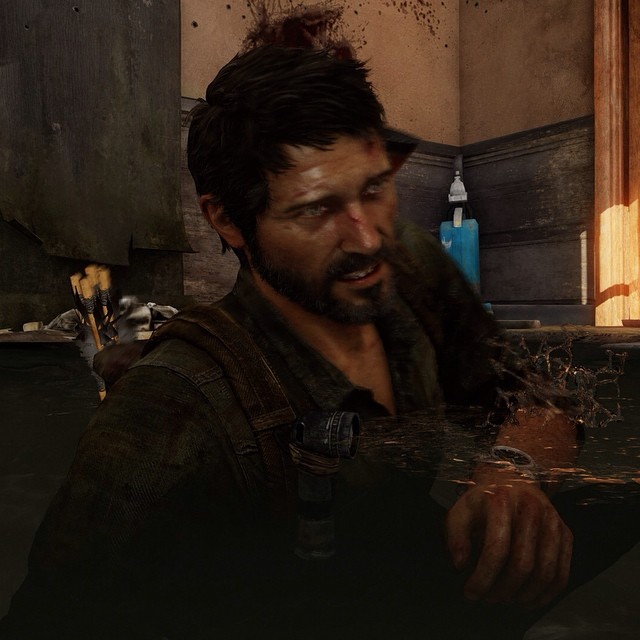This color screenshot from "The Last of Us" video game series features Joel Miller, a middle-aged man with dark hair, a mustache, and a beard. He is captured looking to the right, dressed in a dark-colored shirt with backpack straps visible over his shoulders. Joel has his hand raised, revealing a wristwatch, and there is a noticeable blurring around his arm, the source of which is unclear. Several arrows are protruding from the top of his backpack. The background is a gritty, dilapidated room with dirty walls and yellow curtains hanging at the top right edge. Sunlight filters through the bottom of the curtains, adding a hint of illumination to the otherwise bleak setting.